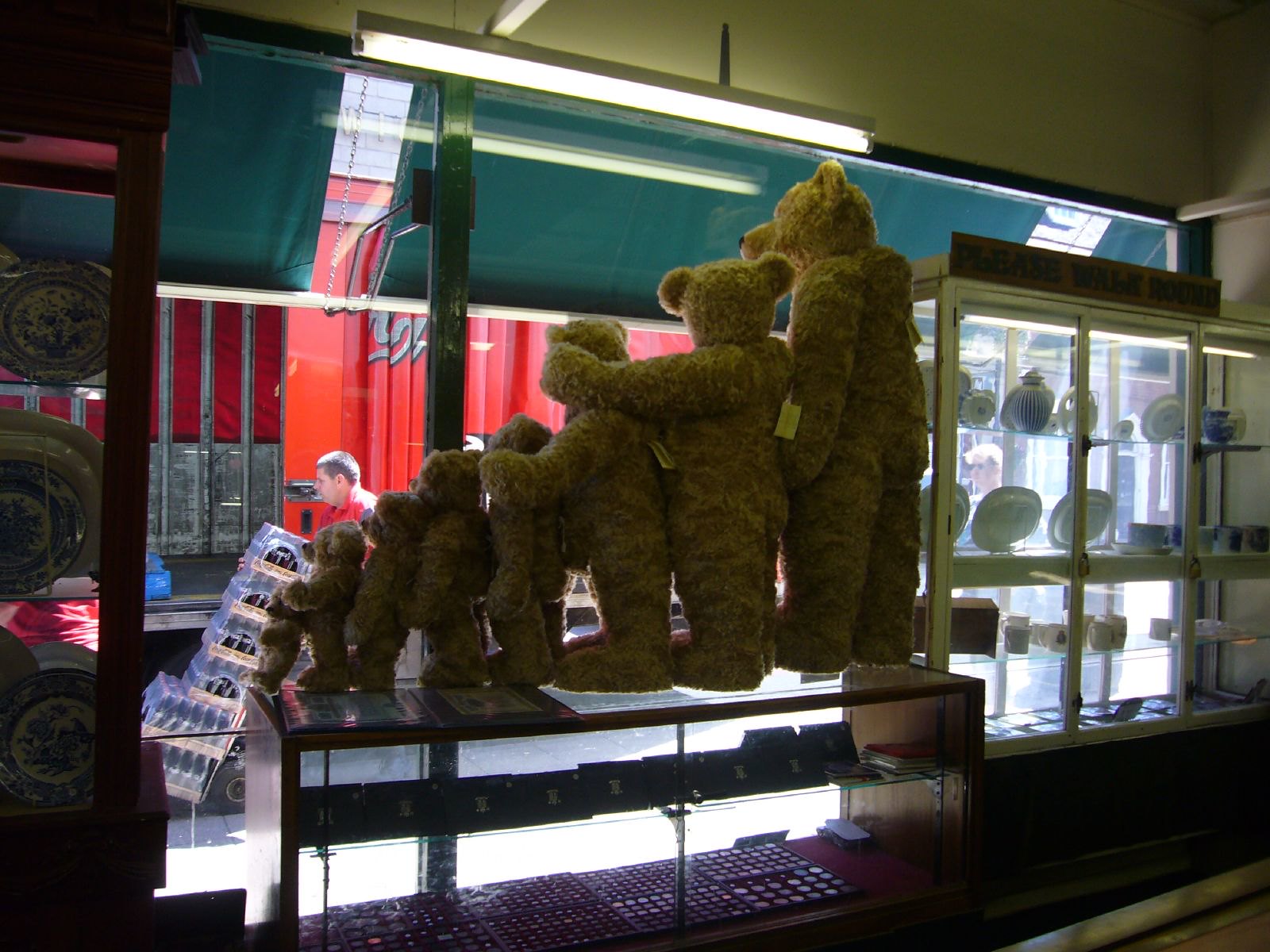This detailed, landscape-orientated photograph captures a storefront view from within an antique shop. At the forefront, atop a low glass display case filled with jewelry, pendants on a red base, and potentially black boxes or watches, stands a line of nine teddy bears. These bears range in size from the smallest, just a few centimeters tall, to the largest, several feet tall, arranged in a cascading manner from left to right. All the bears are either light brown or tan and are posed as if they were human, with some having their arms over the shoulders of the bear in front or leaning back against the larger bear behind them. They are facing towards the right, slightly turned to give the impression of looking out the large window behind them. Beyond the window, a delivery man in a red shirt with short brown hair, is unloading crates from an open red trailer, clearly visible against the daylight. To the right of the bears is a glass shelf with white wooden borders, showcasing three rows of pottery with plates and cups. To the left, a dark brown-bordered glass cupboard displays plates with blue designs. Above, a fluorescent light illuminates the scene. This enchanting composition blends the charm of the teddy bears with the nostalgic allure of the antique shop.